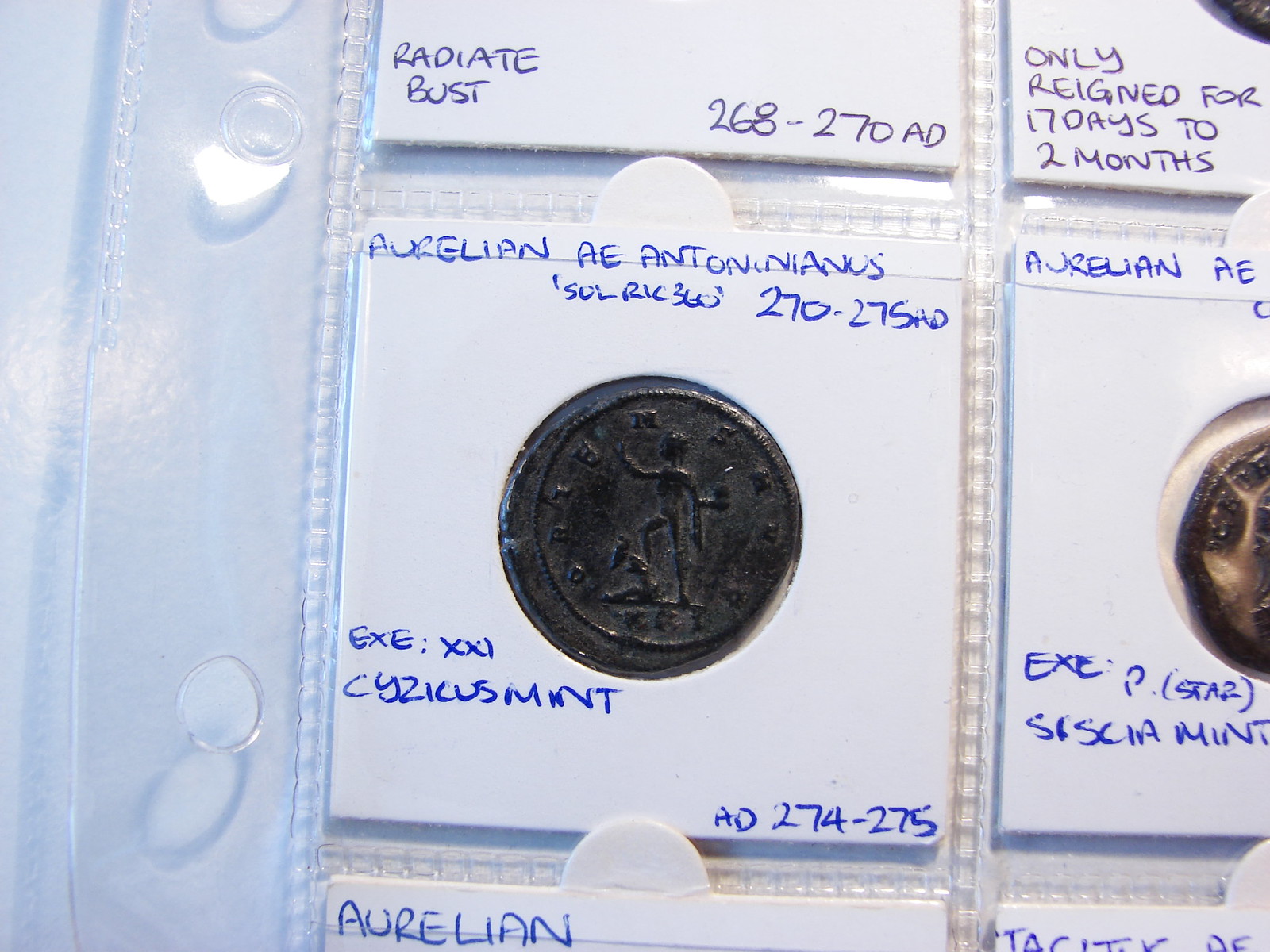The image is a close-up of a meticulously organized coin collection displayed in a three-hole punched plastic binder with individual sleeves. Each coin is securely housed in a white cardboard holder with a clear plastic window, allowing for unobstructed viewing. The featured coin, presented in a weathered, antiquated state, is held in a square-shaped holder with a tab on top for easy handling. Handwritten annotations surround the coin, providing detailed historical context. The prominent coin appears to be an Aurelian A.E. Antoninianus, dating from 270-275 A.D. The inscriptions also note the OLRIC 360 270-275 A.D. and CYZICUS Mint. In the lower-left corner of the holder, there's an 'EX; XXI' notation. The described coin's imagery suggests a striking depiction of an explorer standing on a rock, gazing into the distance. The neighboring slots in the binder are partially visible, hinting at the collection's extensive and organized nature.